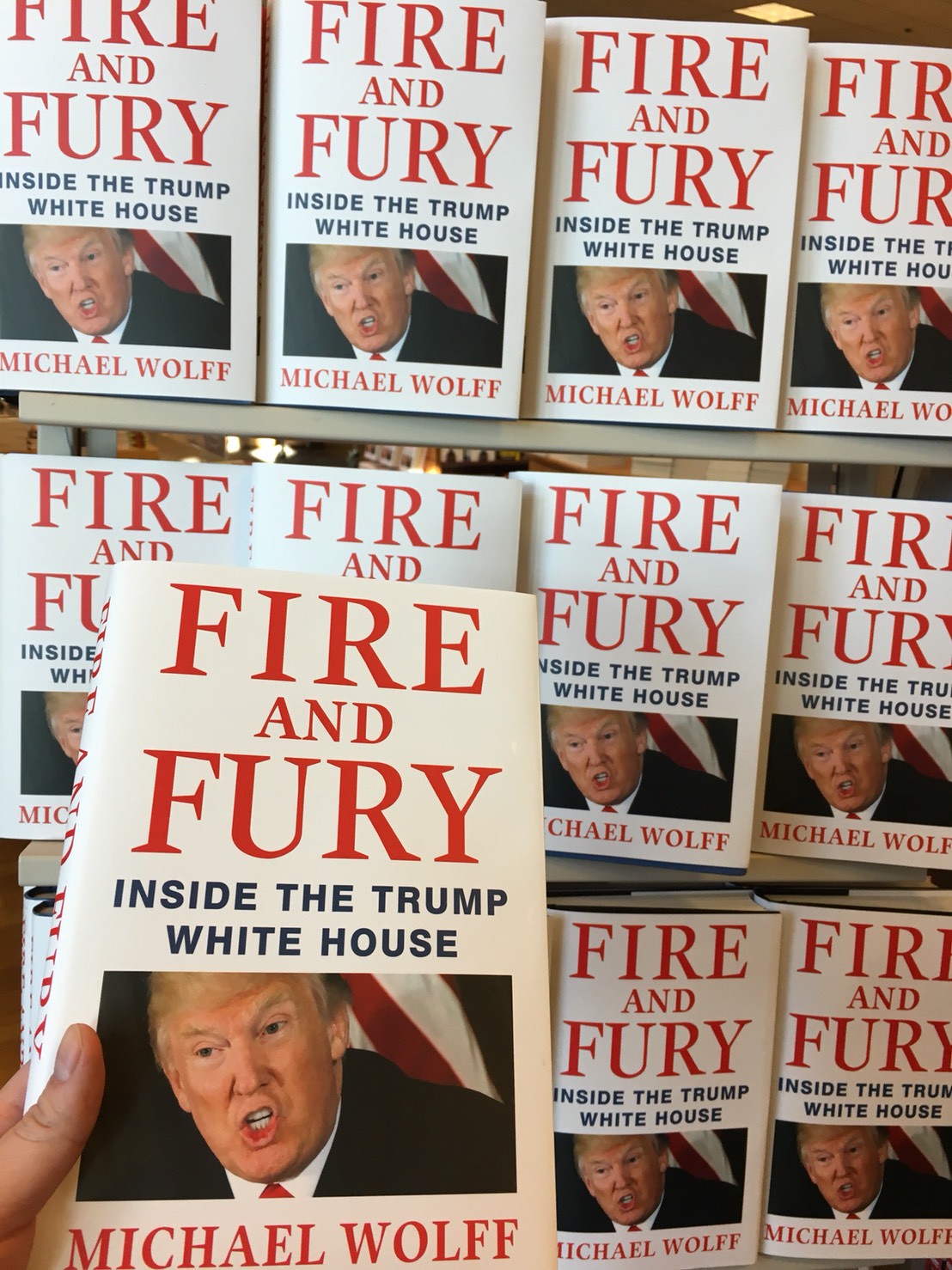The image depicts a display of the book "Fire and Fury: Inside the Trump White House" by Michael Wolff. The display consists of three shelves, each holding four copies of the same book, arranged in rows. The focal point of the image is a person's hand holding up a copy of the book closer to the camera, partially obscuring two copies on the bottom left shelf. This book has a completely white cover with the title "Fire and Fury" prominently displayed in large red capital letters at the top. Beneath the title, in smaller black capital letters, it reads "Inside the Trump White House." Below this text, there is a photograph of Donald Trump, who appears to be making a pursed lip expression, and below the image, the author’s name, Michael Wolff, is written in red caps. The hand holding the book is visible in the bottom left corner of the image, with the thumb and another finger gripping the bottom edge. The other twelve copies of the book sit neatly arranged on the shelves behind.